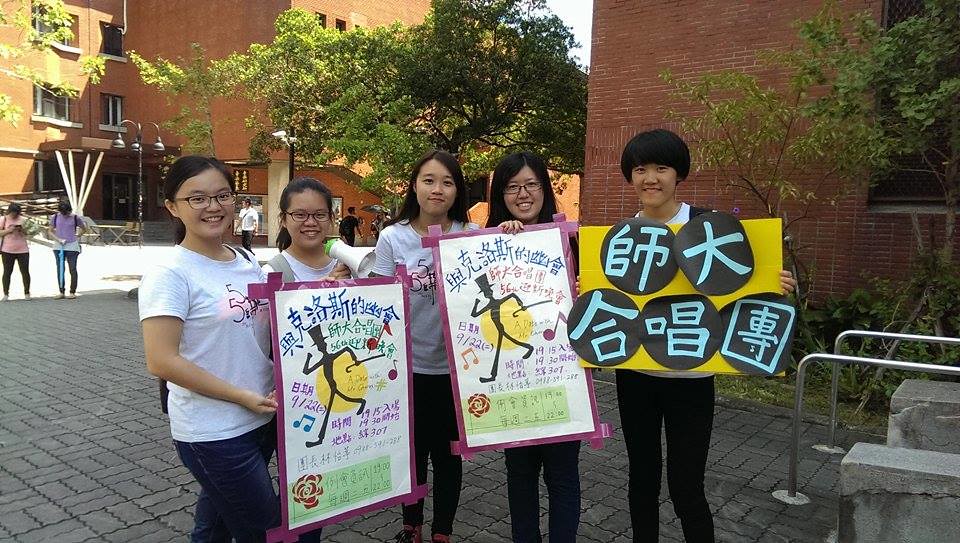This photograph features five young Asian women standing on a gray cobblestone ground in an outdoor area, posing for the camera in front of a red brick building. All five women are wearing white t-shirts and either blue jeans or black pants, and all have dark hair; three of them are wearing glasses. They are holding various placards, which appear to be signs for an event or cause, each featuring different symbols and text in a foreign language, including Chinese characters. One of the signs prominently displays a silhouette of a man holding a baton and includes a yellow circle, while another shows five black backgrounds with light blue Chinese symbols. Behind them, more people can be seen walking around further from the camera. The background also includes several trees adjacent to the brick building, enhancing the outdoor setting of the image.